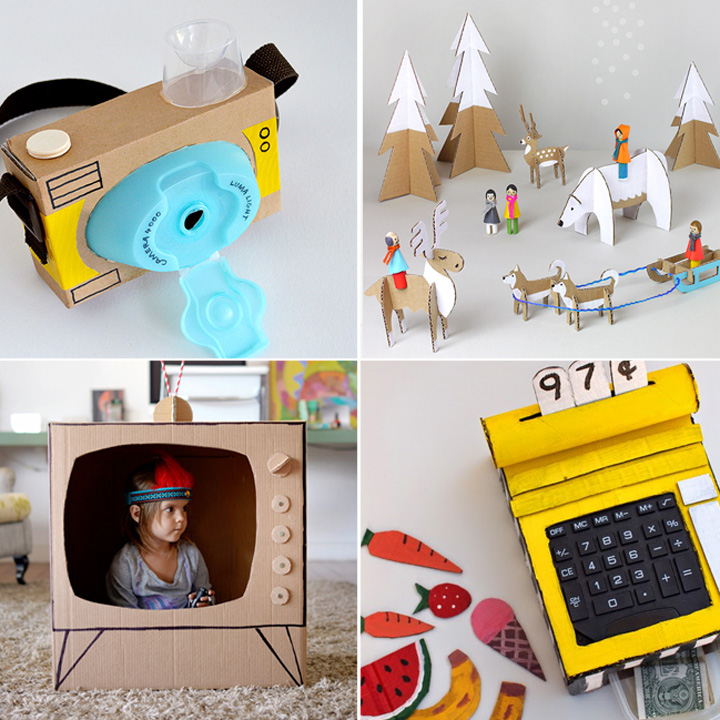The image showcases a creative array of cardboard projects, divided into four sections. In the bottom left, a toddler adorned with an Indian headband sits cheerfully inside a cutout of a retro TV made from cardboard, complete with drawn-on legs and cardboard knobs on the right. Above him in the top left section, there's an intricate cardboard camera featuring a blue plastic lens and a flash made from a plastic cap. The top right section brings to life a wintry scene with cardboard cutouts of snowy trees, a polar bear, a bison, and sled dogs; some hand-painted figures in colorful attire add to the vibrant display. Finally, the bottom right quadrant highlights a cardboard cash register painted in gold and black, cleverly designed with a functional real calculator integrated into the setup. Together, these vignettes celebrate the whimsical and artistic use of everyday materials.